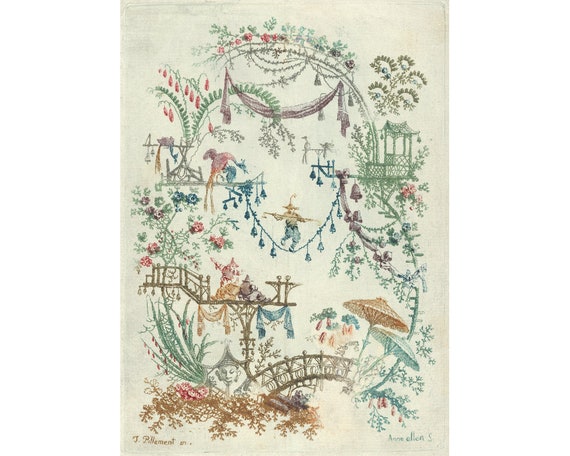The image is a vertically aligned rectangular art print that has the appearance of an aged postcard. The background is a subdued mix of beige and gray with areas resembling stains, contributing to its vintage look. In the lower right corner, a handwritten signature in green reads “Anne Ellen S,” while the lower left corner features “J Bellamont” written in gold. The overall scene is flat with limited depth, yet intricately detailed and whimsical. It features an assortment of natural and man-made elements arranged in a somewhat circular manner around the canvas.

At the base of the image, there is a brown curved bridge and a pier adorned with a straw umbrella. Green ivy and rich teal florals intermingle with pink flowers, creating a lush backdrop. To the lower left, brown leaves can be seen, and leading upward, the scene transitions to include more greenery and a treehouse-like structure.

A man stands balancing on a blue, light-strung rope in the center. He is dressed in blue pants, a brown hat, and holds a brown stick. Above him, a small platform hosts a large bird, and swirled lines and floral motifs fill the upper portion of the image, adding to its dreamlike quality. Green gazebos are also present, blending harmoniously with the rest of the natural elements.